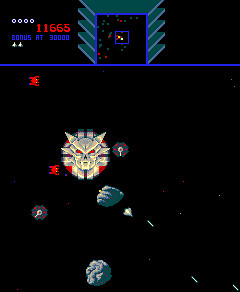The image depicts a video game scene on a black screen featuring various intricate elements. At the top, the red number "11665" is prominently displayed. Below it lies a structure with a royal blue square outline, accompanied by 3D gray layers extending at angles from either side, resembling wings. The square contains multiple blue and red dots, with another smaller blue square inside housing two white dots. A blue line stretches across the screen beneath this structure.

In the middle section of the image, a large, round white demon face on a red background commands attention. The demon, with horns protruding from its ears and glowing red eyes, displays an angry expression. Just below the demonic visage, there's a light blue shape resembling a brain, followed further down by another gray object, also reminiscent of brain matter.